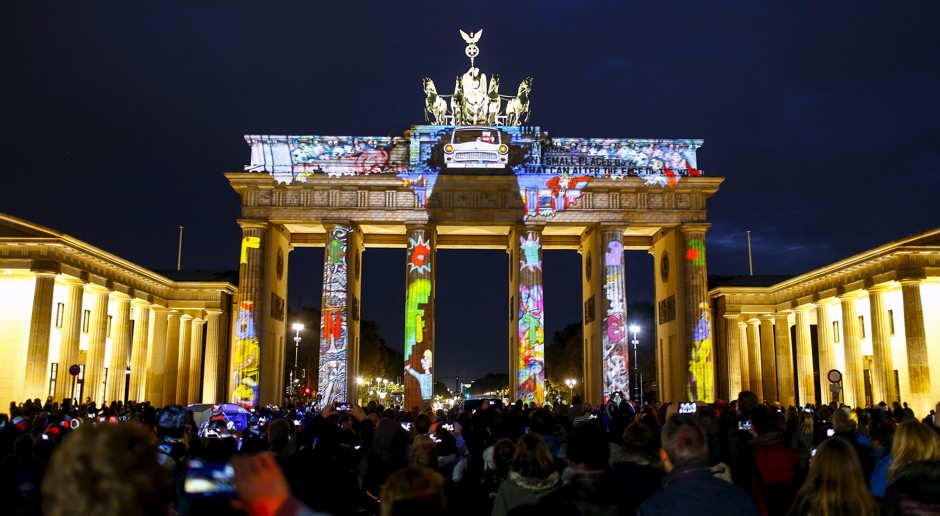This photograph, taken in landscape orientation, captures an outdoor nighttime scene at the Brandenburg Gate in Germany. In the foreground, a large crowd of people holds up their cell phones to photograph or video the spectacle. The gate's classical architecture, featuring imposing white marble columns illuminated by incandescent light, stands majestically in the center, flanked by two-story buildings on either side.

Above the gate, colorful, projected images fill the structure, giving the scene a vibrant, graffiti-like appearance. The projections appear cartoony and even include characters like Bart Simpson. Adding to the surreal ambiance, additional decorative elements such as a car and fake animals are illuminated at the top. Amid the various projections, there is text in English conveying a political message, albeit somewhat obscured. The overall scene creates a juxtaposition of historical grandeur and modern artistic expression, making for a visually striking and culturally layered image.